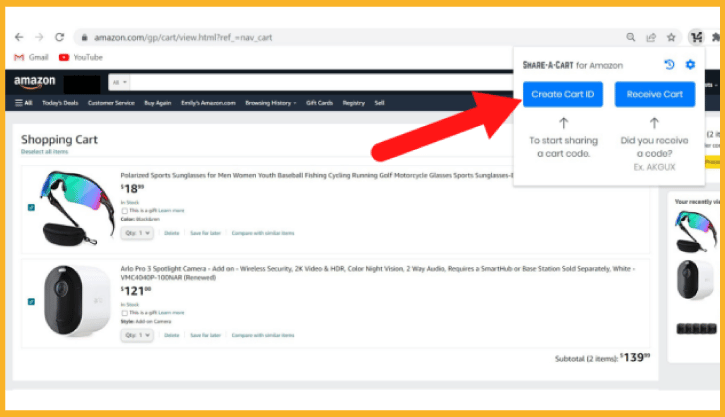An image screenshot shows an Amazon shopping cart page with an orange border. 

At the top of the image, navigation icons are discernible, including a left arrow, a reload button, and various website icons such as Amazon, Gmail, YouTube, and others. The Amazon URL, along with a search bar featuring options like "All," "Today's Deals," and "Customer Service," is clearly displayed.

A prominent red arrow is pointing towards a window on the page titled "Share-A-Cart for Amazon." This window contains instructions for creating a cart ID to share, with options in blue text: "Create Cart ID to start sharing a cart code" and "Did you receive a code?" followed by an example code "EXAKGUX."

Below this section, the shopping cart's contents are detailed. The shopping cart includes items such as "Polarized Sports Sunglasses for Men, Women, Youth" listed with multiple uses including baseball, fishing, cycling, running, golf, and motorcycle. Another item is the "Arlo Pro 3 Spotlight Camera, Wireless Security, 2K Video, HDR, Night Vision, Two-Way Audio, Smart Hub Base Station" noted as "sold separately" for $121. The total for two items in the cart is $139.99.

The surrounding background of the page is mainly white, complemented by an orange border with some gray elements dispersed throughout.